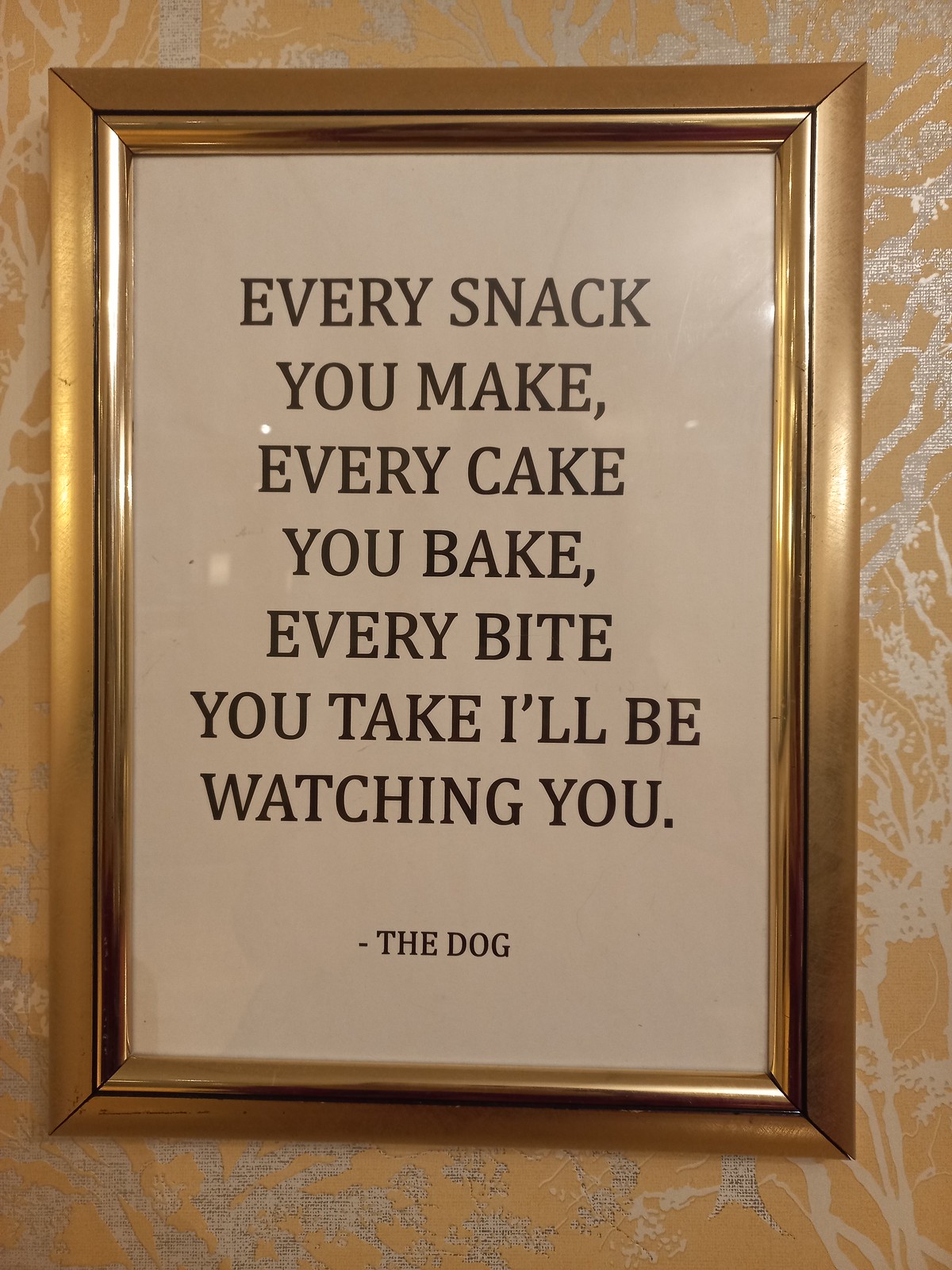The image depicts a humorous quote reminiscent of the Police's song "Every Breath You Take," framed in an ornate golden picture frame. The quote, written in black uppercase lettering on a white background, reads: "Every snack you make, every cake you bake, every bite you'll take, I'll be watching you. - The Dog." The golden frame, which has a shiny appearance, adds to the decor of a wall covered in elaborate gold and silver wallpaper. The wallpaper itself features intricate patterns resembling trees and branches with a slight sparkle where the silver is present. The overall setting contrasts the playful nature of the quote with the luxurious, almost whimsical elegance of the surroundings.